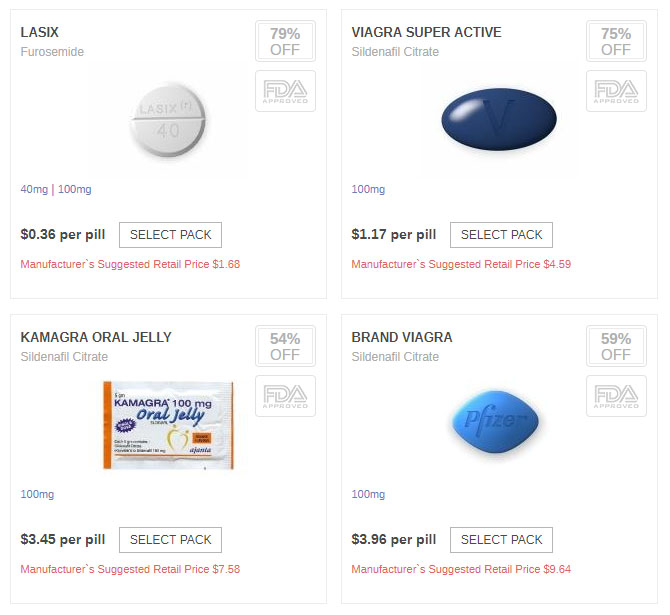The image features a web page against a white background that advertises various medications available for purchase. In the top left corner, there is a section dedicated to Lasix (furosemide). This section includes two highlighted boxes: the first one, situated at the top, displays a "79% off" discount offer, while the one below it indicates FDA approval.

The focal point of the Lasix section is an image of a round, white pill bisected with a horizontal score line. The pill is inscribed with "Lasix 40," denoting its dosage of 40mg. Additional text beneath the pill reads "40mg and 100mg, $0.36 per pill," offering pricing information. Accompanying this is a rectangular "Select Pack" button, promoting the selection of specific quantities for purchase. Below this button, in red text, is the manufacturer’s suggested retail price of $1.68 per pill.

Further down the page, another section advertises Camagra Oral Jelly. This part includes two highlighted boxes: the first offers a "54% off" discount, and the second confirms FDA approval. The details mention that Camagra contains sildenafil citrate with a 100mg potency, priced at $3.45 per pill.